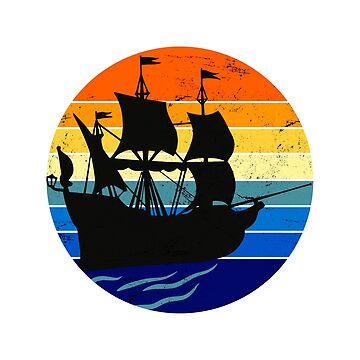The image features a circular design set against a white background. This circle is divided into multiple horizontal color sections, creating a gradient effect. Starting from the top, there's a semicircle of vivid orange, followed by layers of lighter orange, yellow, and lighter yellow. Below these, the colors transition to green, then two distinct shades of blue, with the bottom semicircle composed of darker blue hues interspersed with lighter blue wave patterns.

At the center of this colorful circle is a striking black silhouette of a ship featuring four towering masts. The ship is positioned so that its hull aligns with the blue sections at the bottom, while its sails extend upward across the various colored stripes. The four masts are arranged with two to the right, one in the middle, and one to the left, and a small flag or sail is notably seen on the left side. The contrast between the black ship and the vibrant colors of the background creates a visually compelling and detailed composition.